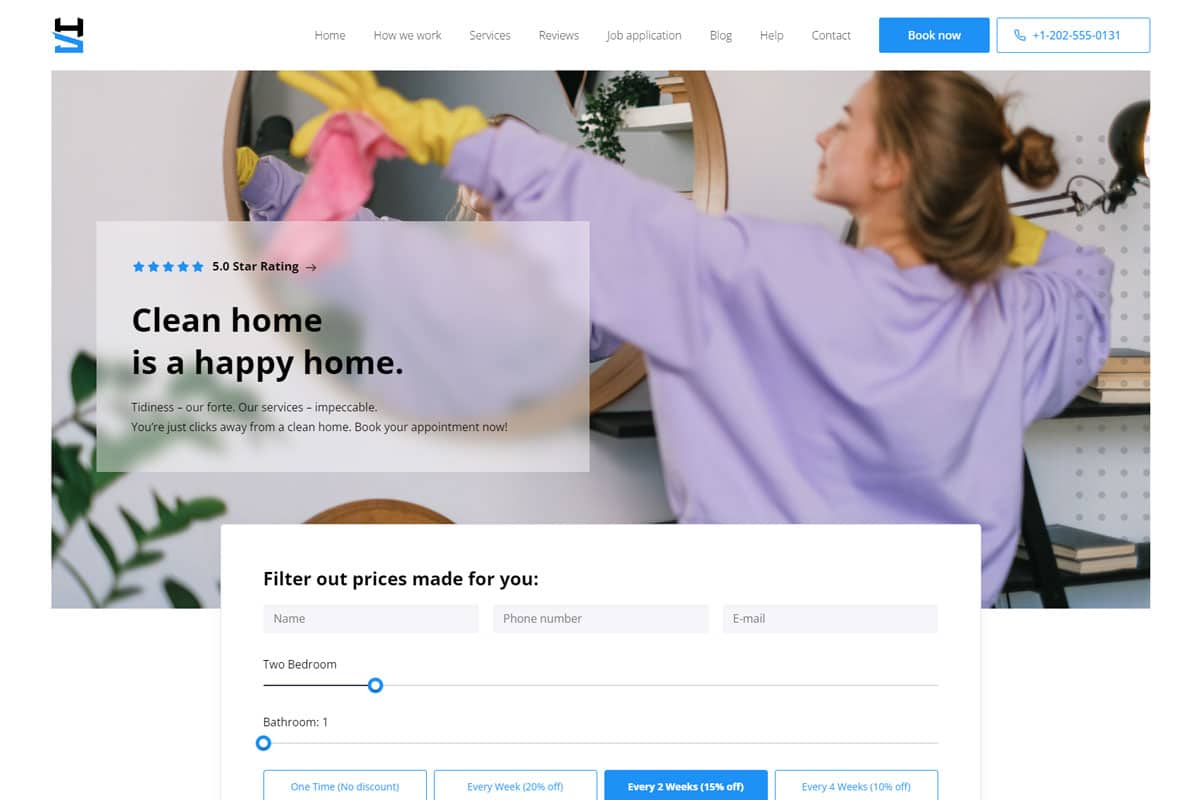In this image, we see a Caucasian woman with light brown hair tied up at the back, wearing a pink top and yellow gloves, holding a pink cloth as she cleans a mirror. The background includes a white wall and bookshelves.

At the top right of the image, there's a white navigation menu featuring gray font and a small blue mark under the 'H' in 'Home'. The menu items are listed from left to right as: Home, How We Work, Services, Reviews, Job Application, Blog, Help, Contact, and Book Now. The 'Book Now' button is highlighted in white font against a blue background. A phone number, (202) 555-0131, is displayed near the top.

In the photo, there's a white box featuring a 5-star rating in blue with an arrow pointing to the right in black, followed by the text "5-star rating" in black font. Below this, the slogan "A clean home is a happy home" is visible. Another line in black font beneath reads, "Tidiness, our forte. Our services, impeccable. You're just clicks away from a clean home. Book your appointment now."

Further down, there's another white box containing the text "Filter out prices made for you." and a gray box below it asking for "Name," "Phone Number," "Email," and the option "Two Bedroom." There's a horizontal line with a blue circle to adjust the number of bedrooms. Another line below, labeled "Bathroom 1," also has a blue circle and a gray line to indicate the number of bathrooms.

Lastly, blue font within boxes details pricing options: "One Time: No Discount," "Every Time: 20% off," "Every Two Weeks: 15% off," and "Every Four Weeks: 10% off."